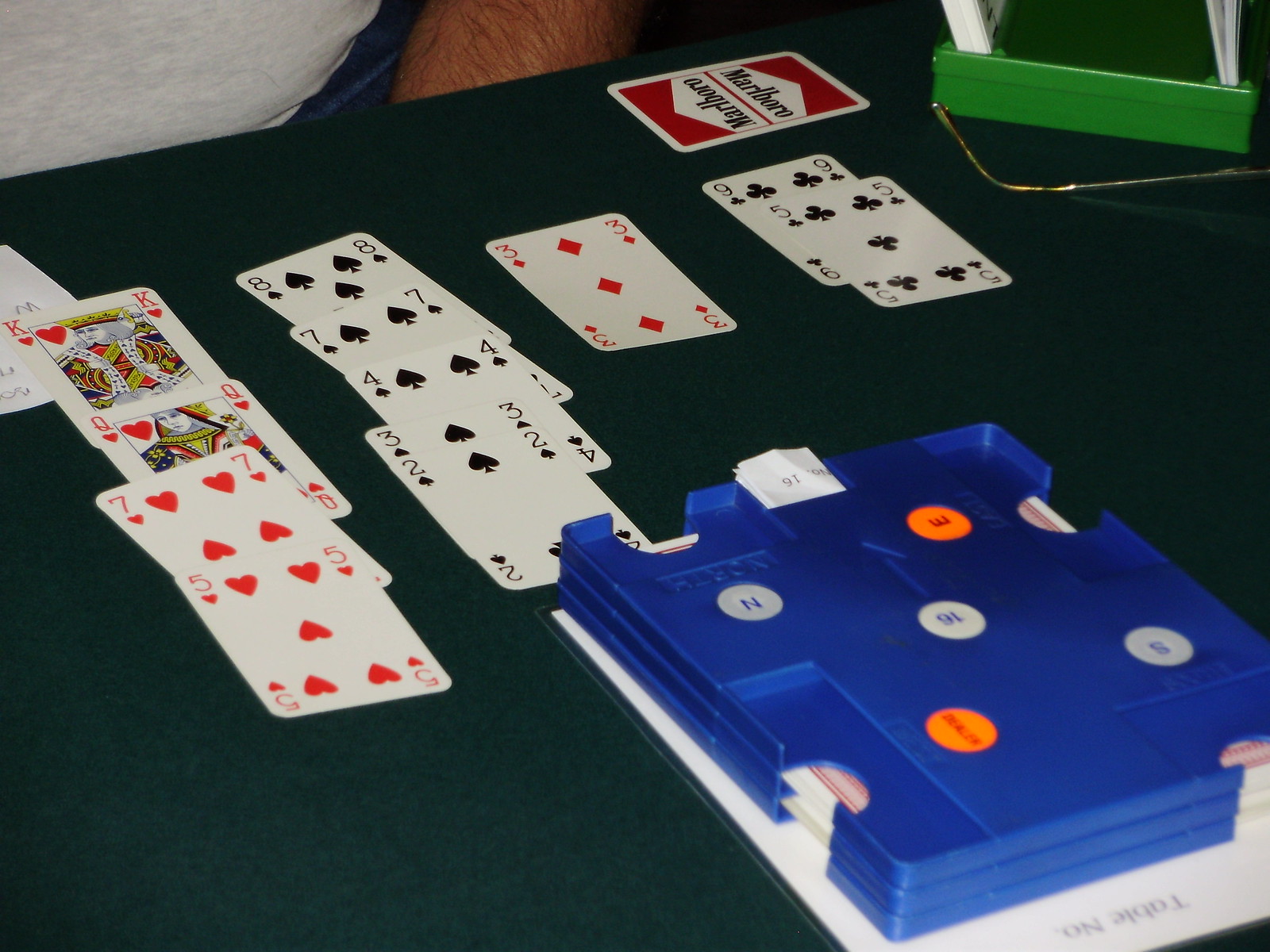The photograph captures a dynamic gaming scene set on a green felt surface, likely that of a gaming table. Dominating the lower right corner is a blue, square-shaped plastic card shuffler, intricately detailed with labels reading "N," "E," "S," and another unreadable label, along with the number "16" prominently centered. The shuffler is loaded with a deck of red playing cards, preparing for action. In front of the shuffler, four cards are meticulously laid out in a diagonal line, the arrangement reminiscent of a solitaire game, with their faces exposed and slightly offset, revealing the card beneath each one. The upper left corner of the image features a partial view of a person dressed in a gray t-shirt and blue jeans. The individual's forearm, tanned and covered in dark hair, adds a human element to the scene, suggesting they are engaged in the card game. The composition of the photograph not only highlights the equipment in use but also hints at the casual atmosphere of a home game.